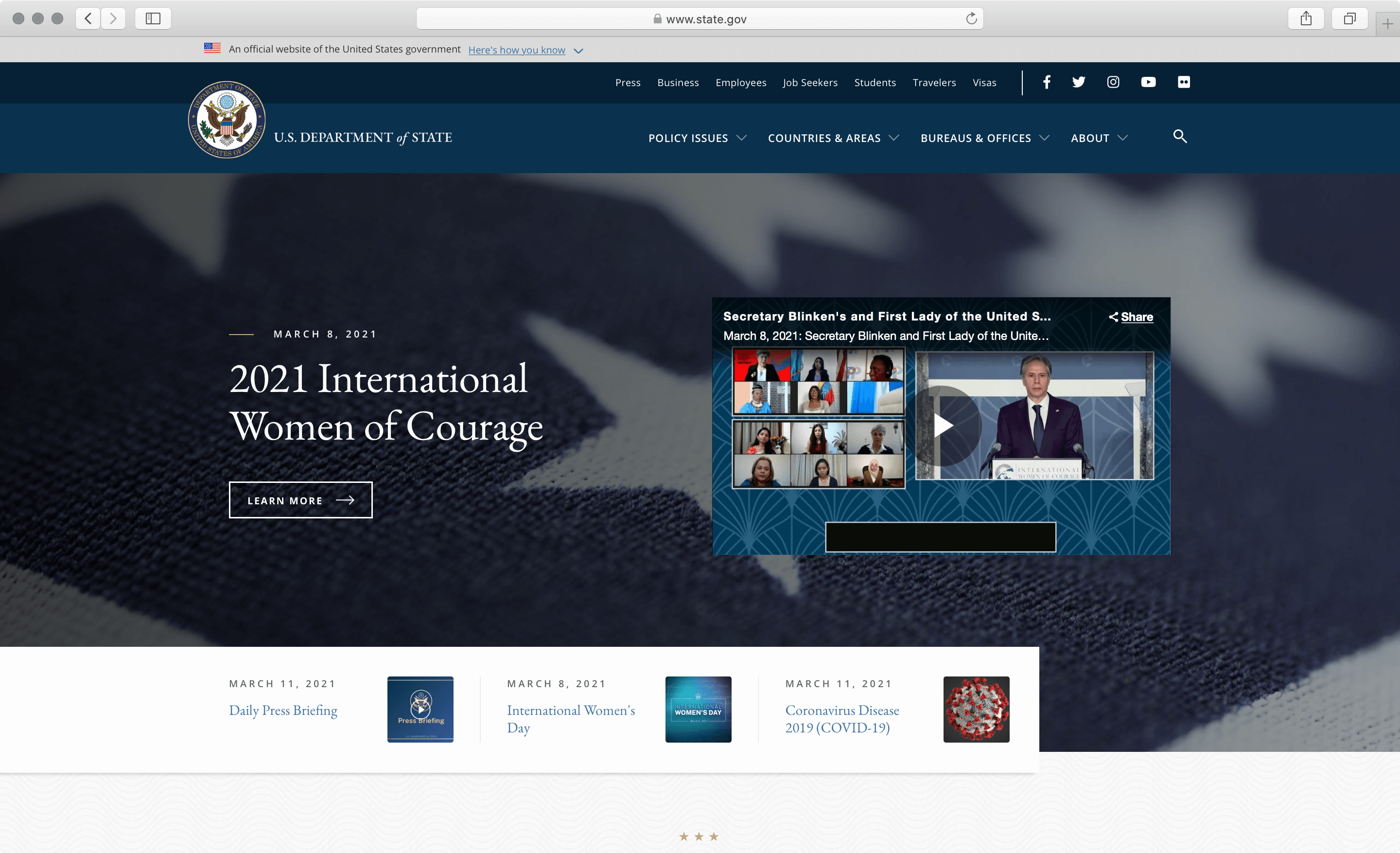The image is a screenshot of a web browser displaying a government website, specifically the U.S. Department of State's homepage. 

At the top left of the browser, there are three gray circles. To their right, navigational icons include a left arrow, a right arrow, and a square box. In the middle top section of the browser is the URL bar which displays "www.state.gov." To the right of the URL bar is the refresh icon, depicted as an arrow going in a circle.

Focusing on the webpage content, the top left of the site features the text "U.S. Department of State" beside the department's logo, which appears to be an eagle. To the right of this logo are categorized links: "Policy Issues," "Justices," "Bureaus and Offices," followed by a bell icon. Further right is a white magnifying glass icon, indicating a search function.

At the very top right corner, social media icons for Facebook, Twitter, Instagram, and YouTube are displayed. 

In the main content area, prominently to the left, is the text "2021 International Woman of Courage," with a "Learn More" button below it, enclosed in a box.